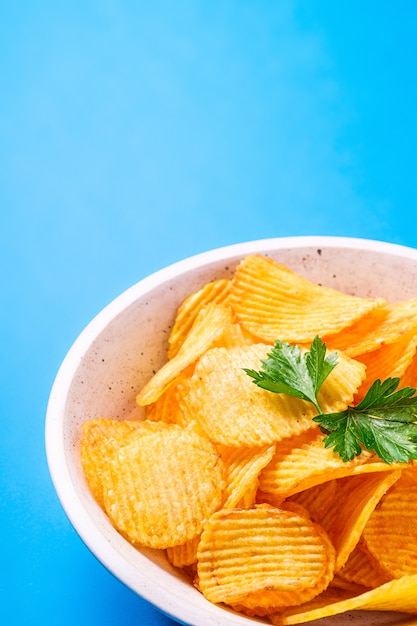This image showcases a bright and eye-catching photograph of a bowl of ruffled potato chips. Dominated by an almost neon aqua blue background, the rectangular photo features the long sides on the left and right, and the short sides on the top and bottom. Positioned in the bottom right corner, the bowl, though partially cut off, reveals about three-quarters of its form. It's a white ceramic bowl with black speckles, appearing slightly pale pink under certain lighting. The bowl is brimming with crispy, brightly orange, ruffled chips, likely barbecue-flavored due to their reddish hue. Adding a touch of elegance, two small, bright green parsley leaves rest atop the chips, contrasting beautifully with the golden potato color. The image captures the light shining from above, emphasizing the texture and sheen of both the chips and the herbs.